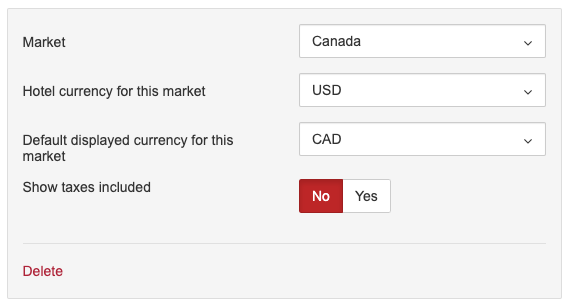This image displays a detailed screenshot of a payment settings interface on a light grey background. A white border surrounds the entire image. 

On the left side, the word "Market" is prominently displayed in black text. Adjacent to it is a white dropdown box containing the word "Canada" in black lettering, accompanied by a down-arrow symbol indicating that more options are available.

Directly below this, the phrase "Hotel Currency for this Market" is written in black text. To its right, a white search box is visible with "USD" selected, and another dropdown arrow for currency options.

Further down, the text "Default Displayed Currency for this Market" appears on the left in black. Next to this is a white search box with "CAD" highlighted, showing that it is the selected option. It also features a dropdown arrow to the right for changing the currency.

The next line of text, "Show Taxes Included," is placed on the left in black. To the right of this text, a toggle box shows two options: "No" and "Yes." The "No" option is highlighted in red with white lettering, indicating the current selection, while "Yes" remains unselected in white with black text.

Below these settings, a thin grey line separates the toggle options from the final element. At the bottom left corner of the interface, the word "Delete" is displayed in red text, potentially indicating a feature to remove settings or configurations.